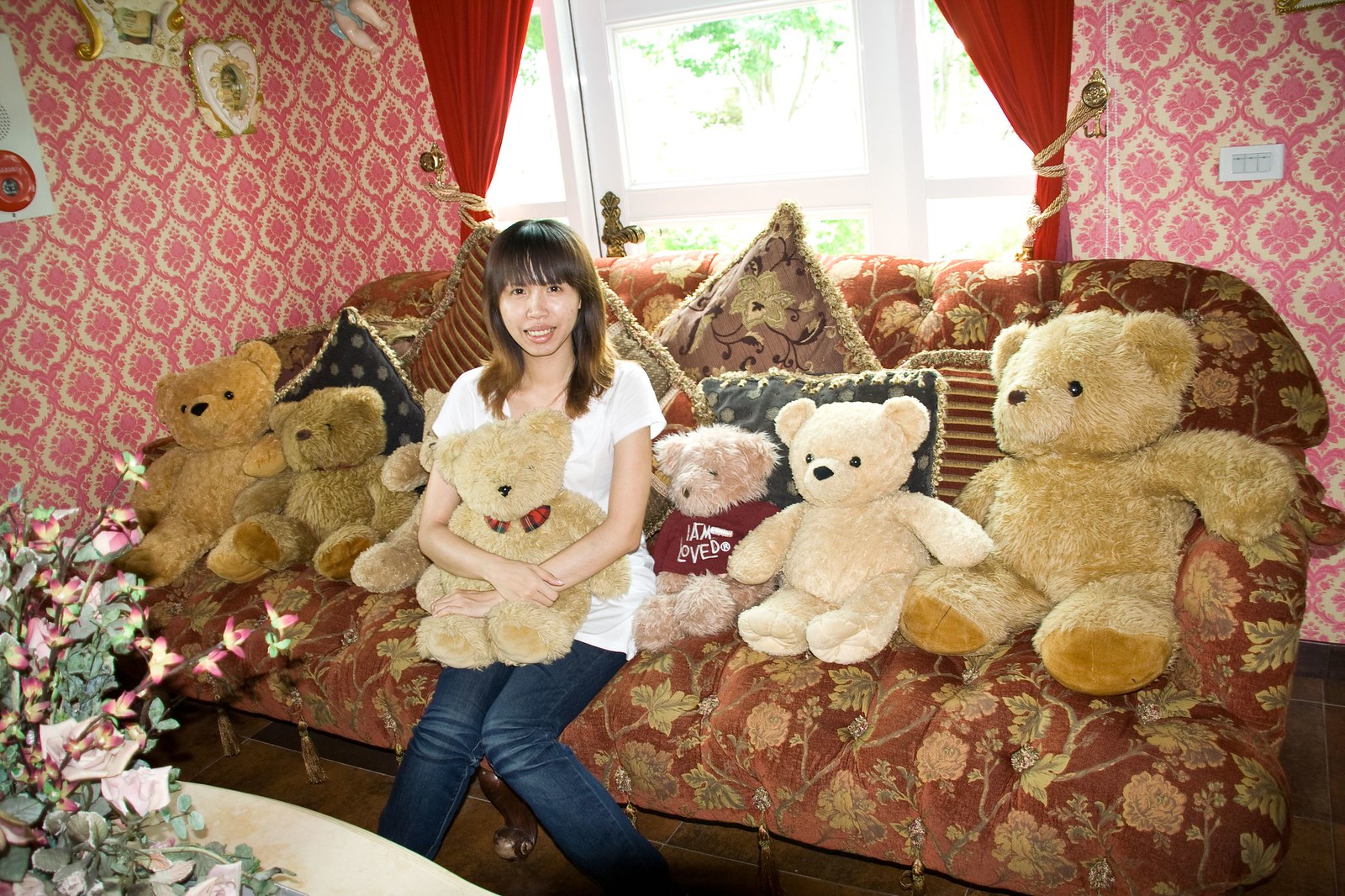The image depicts a cheerful Asian woman in her late teens or early twenties, sitting in the center of a long, rusted burnt-orange couch adorned with intricate floral patterns. She is holding a light brown teddy bear featuring a plaid bow in black, green, and red. The woman, who has bangs and brownish-blonde shoulder-length hair, is dressed in a white short-sleeved blouse and blue denim jeans. Flanking her on either side are six teddy bears of varying sizes and shades of brown, one of which wears a burgundy shirt emblazoned with the words "I am loved." The couch is further accessorized with an array of throw pillows in different patterns, augmenting the room's overall eclectic style.

In front of her sits a table with a vivid floral display, complementing the pink and green bouquet seen nearby. The backdrop is a visually striking wall covered in pink patterned wallpaper, which adds to the room's multitude of motifs. Behind the couch is a white-framed window allowing ample sunlight to stream in, framed by red curtains tied back with rope, enhancing the room's warm, inviting ambiance. The combination of detailed patterns, from the floral couch and pillows to the wallpaper, along with the charming collection of teddy bears, creates a cozy, whimsical setting.